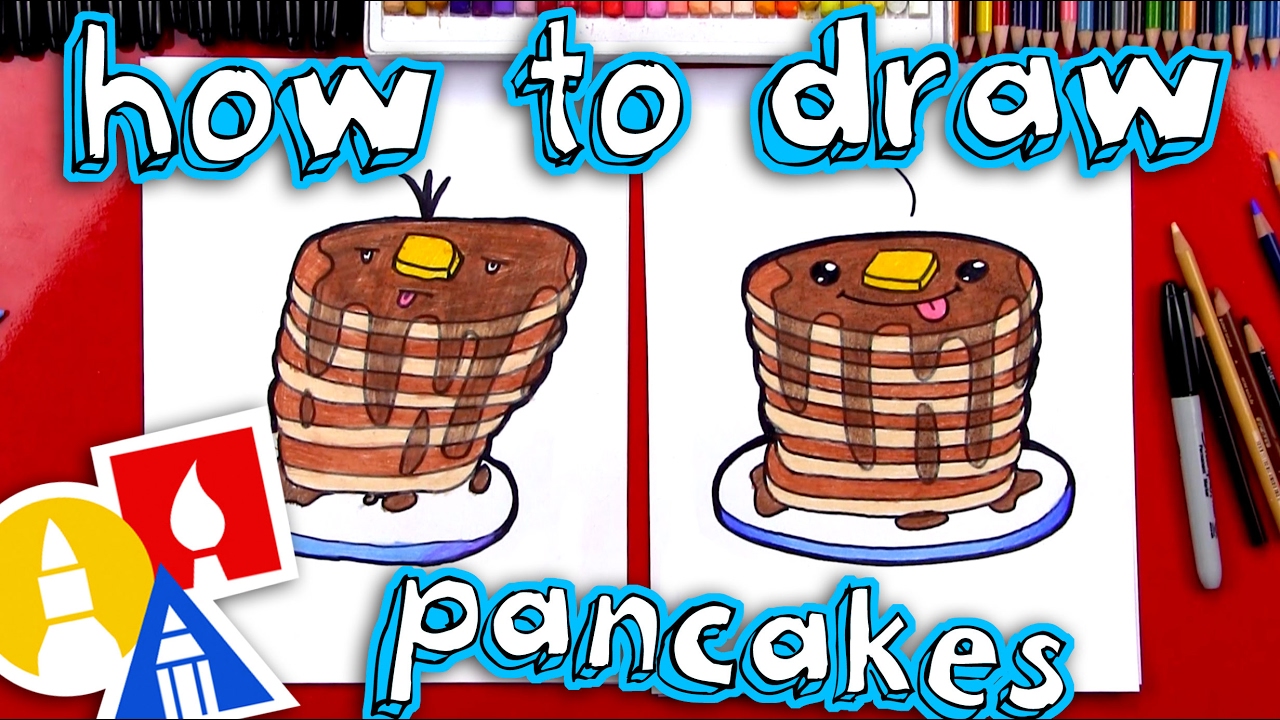This image appears to be a still frame from a YouTube tutorial titled "How to Draw Pancakes," displayed in bright white letters with a blue outline. The scene is set on a red table or desk, cluttered with various art supplies, including a black Sharpie, colored pencils, and markers. 

At the top of the image, there's a lineup of drawing instruments, with black-capped markers on the upper left and a case of colorful markers centrally placed. A strip of colored pencils can be seen on the upper right.

In the center of the image are two A4-sized pieces of paper, each featuring a cartoon drawing of a stack of pancakes on a white plate with a blue border. The pancakes are a light brown color, drizzled with syrup and topped with a pat of butter, which serves as the nose for the pancake faces. The pancake on the left appears less neatly drawn, leaning slightly to the right and featuring black eyes, a smile, a tuft of brown hair, and a pink tongue. The pancake on the right, likely the demonstration version, is more polished, with large white eyes and a big smile with its tongue sticking out.

Overlaying the image are the words "How to Draw Pancakes" in a hand-drawn style font, with the heading "How to Draw" at the top and "Pancakes" at the bottom. In the lower-left corner, three icons are visible: a red square with a white paintbrush, a yellow circle with a white marker tip, and a blue triangle with a white pencil.